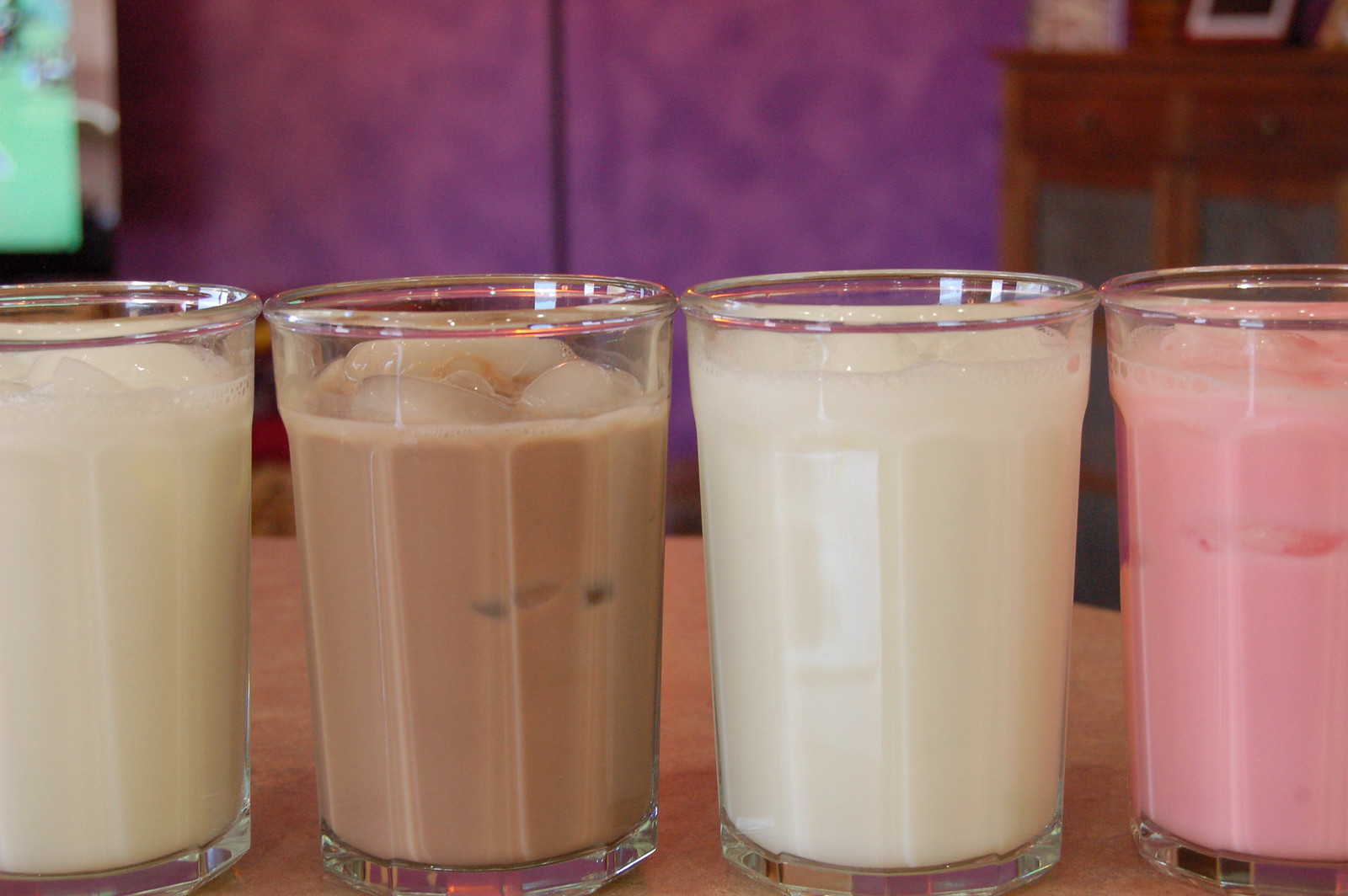This detailed image depicts four clear, shiny, bubbled glasses filled with different types of milk, each containing ice cubes. Arranged in a row on a light brown tabletop, the glasses feature a variety of colors: the first and third glasses contain creamy white milk, the second glass holds chocolate milk, and the fourth glass is filled with a very vibrant pink strawberry milk. Notably, the chocolate milk appears to have been drunk the most, with the level being slightly lower than the others by about half an inch. In the background, there's a blurred scene featuring a purple wall, a wooden shelf, a brown piece of furniture, and a barely visible green spot possibly indicating a window view. Despite these background details, the four distinct glasses of milk remain the clear focal point of the photo.